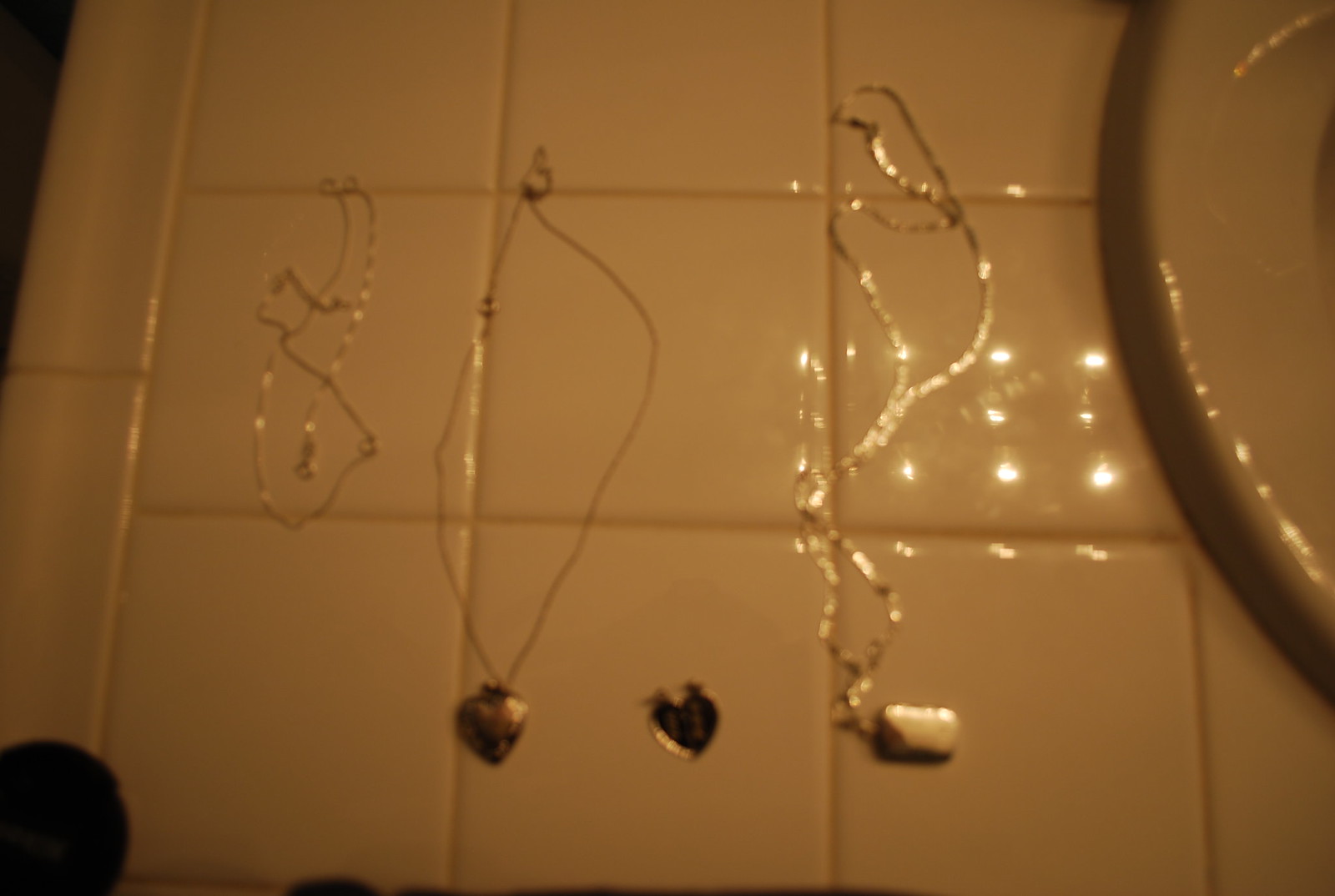The image is a blurry, glary color photograph taken in a bathroom, capturing a white ceramic tile countertop with a partially visible rim of a porcelain sink on the right side. On the countertop, there are four pieces of jewelry, all gold or gold-colored. The first item is a thin gold chain without a pendant. The second is a gold chain with a heart-shaped locket. Beside it lies a separate gold heart pendant, possibly from the broken locket. The last piece is a longer gold chain with a rectangular, possibly pillbox-shaped locket. An overhead light fixture with multiple small lights is reflecting off the glossy tiles, adding to the glare and reducing the clarity of the image.